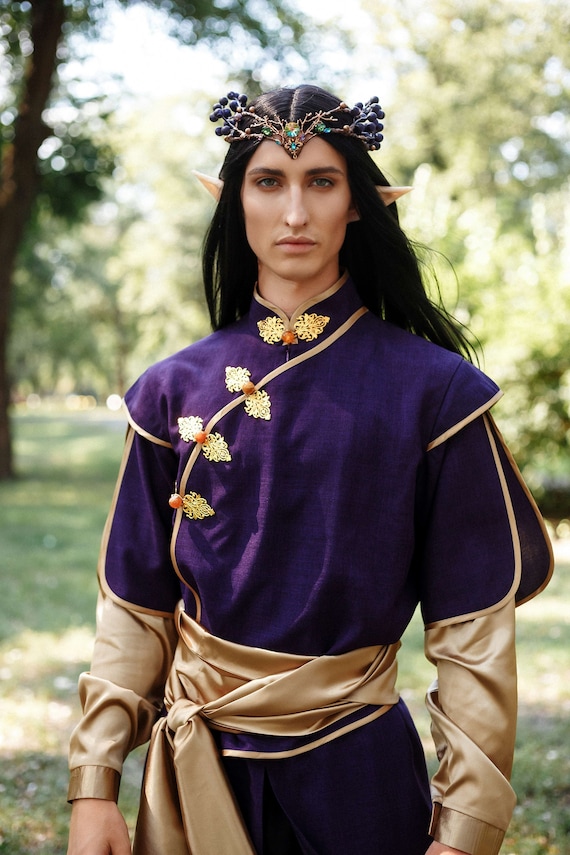This is a detailed photograph of a man dressed as an elf, possibly for cosplay. He has long, dark black hair flowing down his back and piercing blue eyes set beneath thick, well-groomed eyebrows. His strong chin and full lips add to his distinguished and handsome appearance. His elf attire includes long, pointed ears that jut prominently from each side of his head.

The man is adorned in a rich, purple tunic with intricate gold sleeves and a matching gold sash wrapped around his waist. The tunic features tiered sleeves that alternate in length, revealing a champagne-colored layer underneath. Decorative brooches secure the neckline and run up one side of his chest, joined by small orange buds resembling buttons. His outfit includes a short-sleeved shirt worn over a long-sleeved gold garment, the gold cufflinks peaking from beneath the layers.

On his head, he wears a remarkable crown, designed to look like metalwork branches, possibly adorned with fruits and berries. It features blue and bluish-green gemstones, some resembling blueberries, incorporated into its intricate design. The crown's centerpiece dips slightly into his forehead, adding to the regal and otherworldly impression.

The photograph is set against a blurred background of light green and yellow hues, suggesting a sunlit forest or park. The combination of professional lighting and the serene outdoor setting enhances the subject's ethereal aesthetic, making for a very striking and well-crafted image.